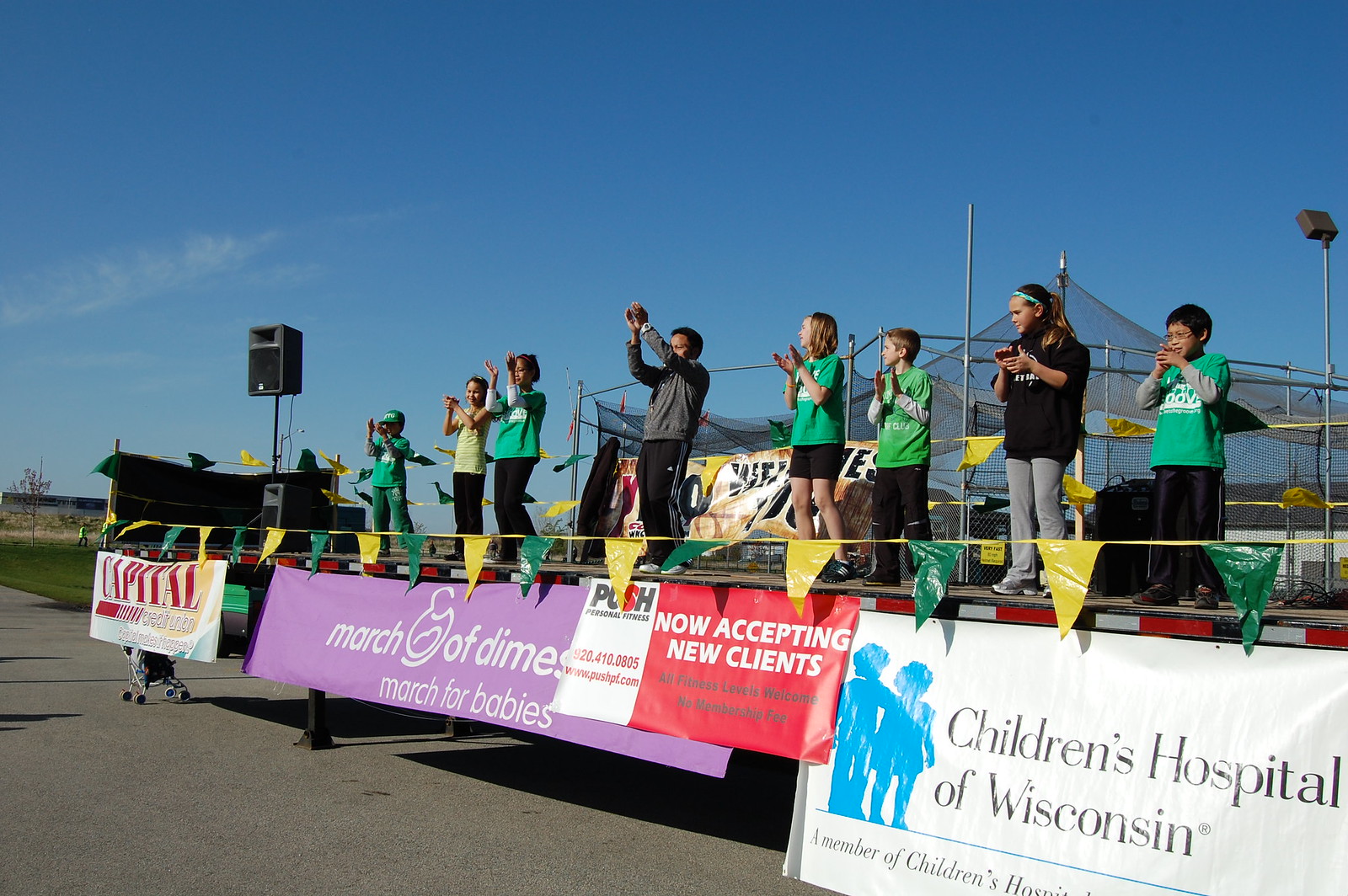The photograph captures an outdoor event set up on a paved gray road, with a green field and a batting cage-like structure in the background. On a raised, portable stage, erected possibly from a truck and set on jacks, nine people are gathered. Seven children in green shirts and black pants or shorts, and two adults, one of whom is centrally positioned and wearing a gray long-sleeved shirt with black pants. All participants are clapping, and it appears they may be performing or singing. 

The front of the stage is adorned with yellow and green triangular pennant banners, and multiple signs. A prominent purple and white banner reads "March of Dimes, March for Babies," and to its right, another sign for "Children's Hospital of Wisconsin, now accepting new clients," in red and white. Speaker equipment is placed at the ends of the stage. The sky above them is clear and blue, with a few wisps of white clouds visible to the left, adding to the cheerful, lively atmosphere of the event.